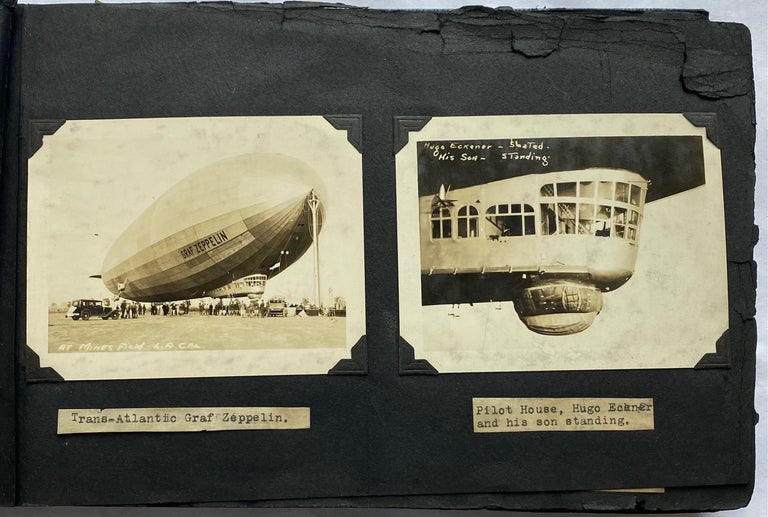This is a set of two sepia-toned photographs mounted on an aged, black photo album page, secured with vintage triangular photo corners. Both photographs are likely historical records of the Graf Zeppelin. The photo on the left prominently features the massive transatlantic Graf Zeppelin airship grounded, capturing its sheer scale and the people standing beneath it, resembling an early automobile's era. Underneath this photograph is a white label with black text reading "Transatlantic Graf Zeppelin." The photograph on the right provides a closer view of the airship, focusing on the passenger windows and the pilot house located beneath the body of the Zeppelin. The upper left corner of this image contains a white text label stating "Hugo Eckener and his son standing," identifying figures associated with the airship, although the individuals are not visible. Despite the photograph's aging sepia tones, the visual details indicate that these images are meticulously preserved to document the significant historical presence of the Graf Zeppelin and its operators.